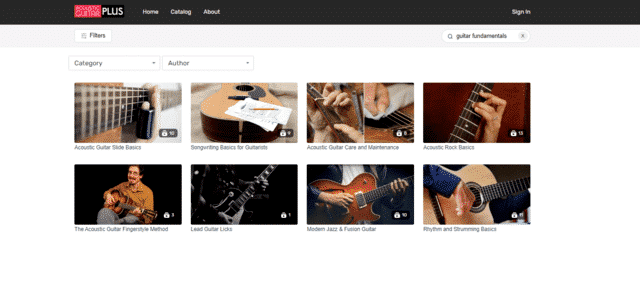This is a detailed screenshot from the Guitar Plus application. At the top of the interface, there is a navigation bar featuring options for 'Home,' 'Catalog,' 'About,' and a 'Sign In' button located in the top right corner. Below this, there is a secondary bar that includes filtering options and a search bar, followed by two dropdown menus labeled 'Category' and 'Author.'

Displayed on the screen are eight videos organized into two rows. The first row of videos includes:
1. "Acoustic Guitar Slide Basics"
2. "Songwriting Basics for Guitarists"
3. "Acoustic Guitar Care and Maintenance"
4. "Acoustic Rock Basics"

In the second row, the following videos are displayed:
1. "The Acoustic Guitar Fingerstyle Method"
2. "Lead Guitar Licks"
3. "Modern Jazz and Fusion Guitar"
4. "Rhythm and Chamming Basics"

Each video is accompanied by an illustrative thumbnail, providing a visual summary of the content offered in this educational and engaging guitar-centric catalog.